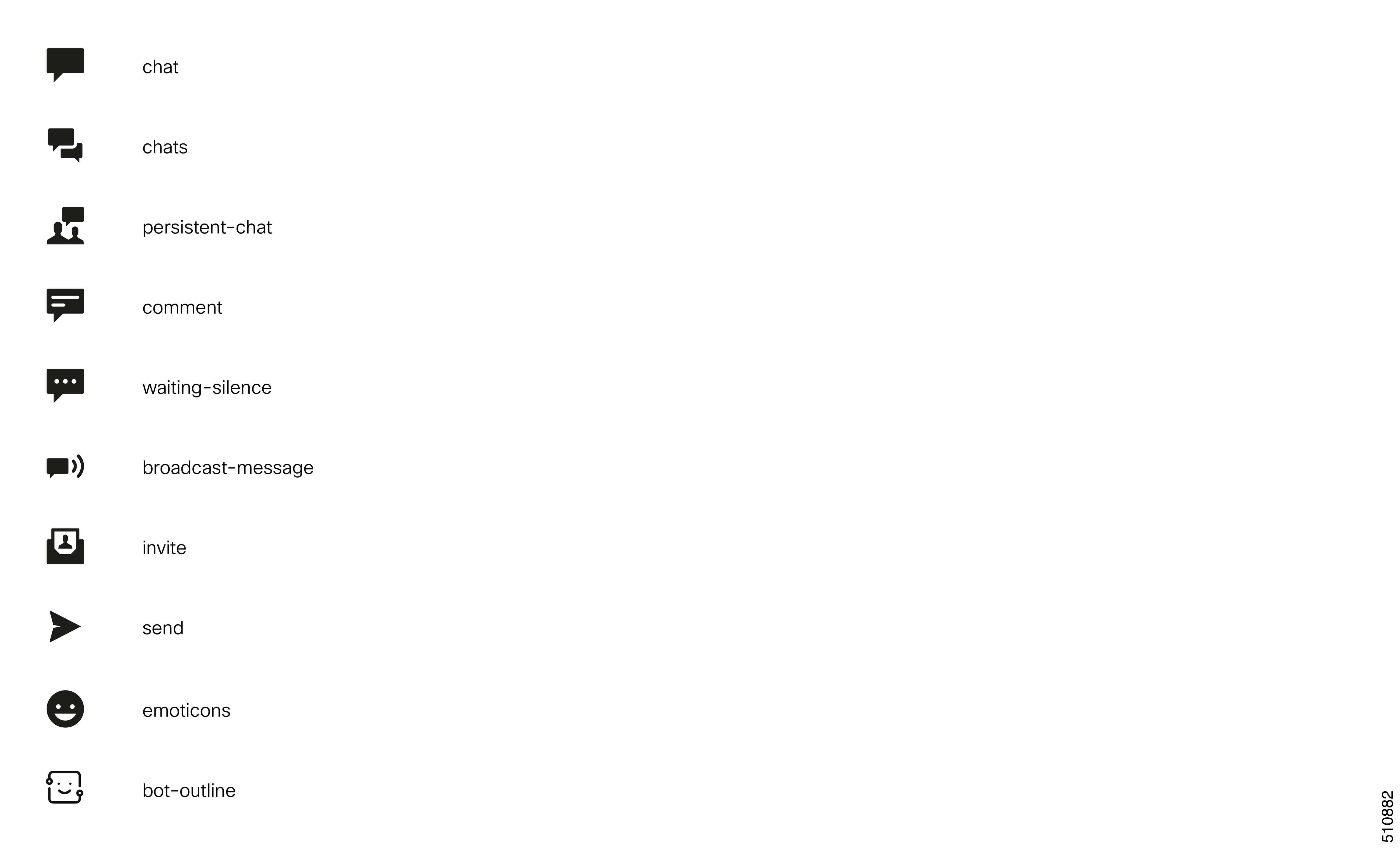A screenshot under the "websites" category displays a minimalist interface featuring a blank white page with a vertical list of ten items on the left side. Each item on the list is accompanied by a small, representative icon. The icons and text are all in black against the white background, creating a stark contrast. Here is a detailed breakdown of the items in the list:

1. **Chat** - Accompanied by a chat bubble icon.
2. **Chats** - Represented by an icon depicting multiple chat bubbles.
3. **Persistent Chat** - Featuring a chat bubble with a pin or anchor symbol.
4. **Comment** - Displayed with an icon of a comment bubble.
5. **Waiting - Silence** - Illustrated by an icon perhaps depicting a clock or hourglass.
6. **Broadcast - Message** - Comes with an icon resembling a loudspeaker or megaphone.
7. **Invite** - Shown with an icon that might look like a plus sign or user silhouette with a plus.
8. **Send** - Represented by a typical email send arrow.
9. **Emoticons** - Illustrated by a classic smiley face.
10. **Bot - Outline** - Accompanied by an icon likely resembling a robot or automation symbol.

Each icon is designed to visually align with its corresponding text, providing a clear and user-friendly navigation menu.